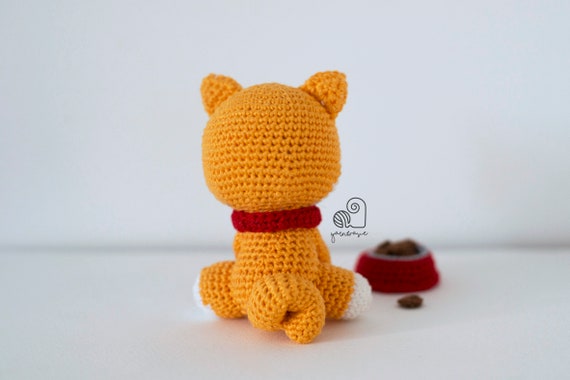This image showcases a crocheted plush cat with its back facing the camera. The cat is primarily orange, featuring small pointed ears, a long curled tail, and small white feet. It wears a red collar around its neck. In front of the cat sits a red crocheted food dish filled with brown crocheted kibble. The cat is positioned on a white surface against a white background. Additionally, a heart-shaped logo with yarn can be seen to the right of the cat in the image.